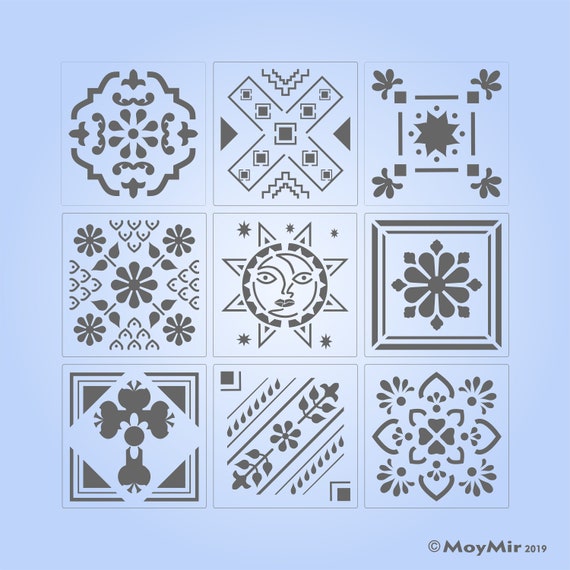The digital art piece showcases nine black and white geometric designs with a floral theme, arranged in a 3x3 grid against a solid blue background. Each square features unique, simplistic artwork, including various floral patterns, crosses, and diamond shapes. The central fifth image prominently displays a whimsical sun with eyes, a nose, and a mouth, surrounded by small stars. The artwork is credited to Boy Mayer and marked with the year 2019.